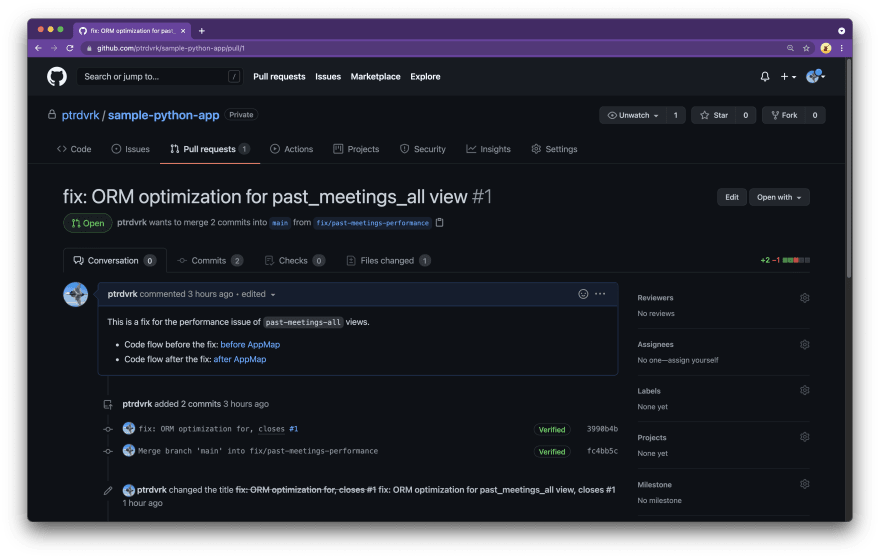The image depicts a screenshot of a GitHub web page with a black background and various textual elements. At the very top, a purple taskbar displays the URL "github.com," indicating the website. The browser's search bar contains placeholders like "search or jump to," "pull request," "issues," "marketplace," and "explorer."

Beneath the taskbar, the title "sample-python-app" appears in blue text against the black background. Further down, a white text description reads, "fix ORM optimization for past_meetings_all view #1." Below this description, there is information about a pull request: "PTR DVRK wants to merge 2 commits into SAIS from fix-past-meetings-performance."

Following this, there is an open conversation box with a comment: "PTR DVRK commented 3 hours ago: This is a fix for the performance issue of past meetings all views." Within this comment, the phrases "Code flow before the fix" and "Code flow after the fix" are also visible, indicating a comparative analysis of the code's performance before and after the proposed changes.